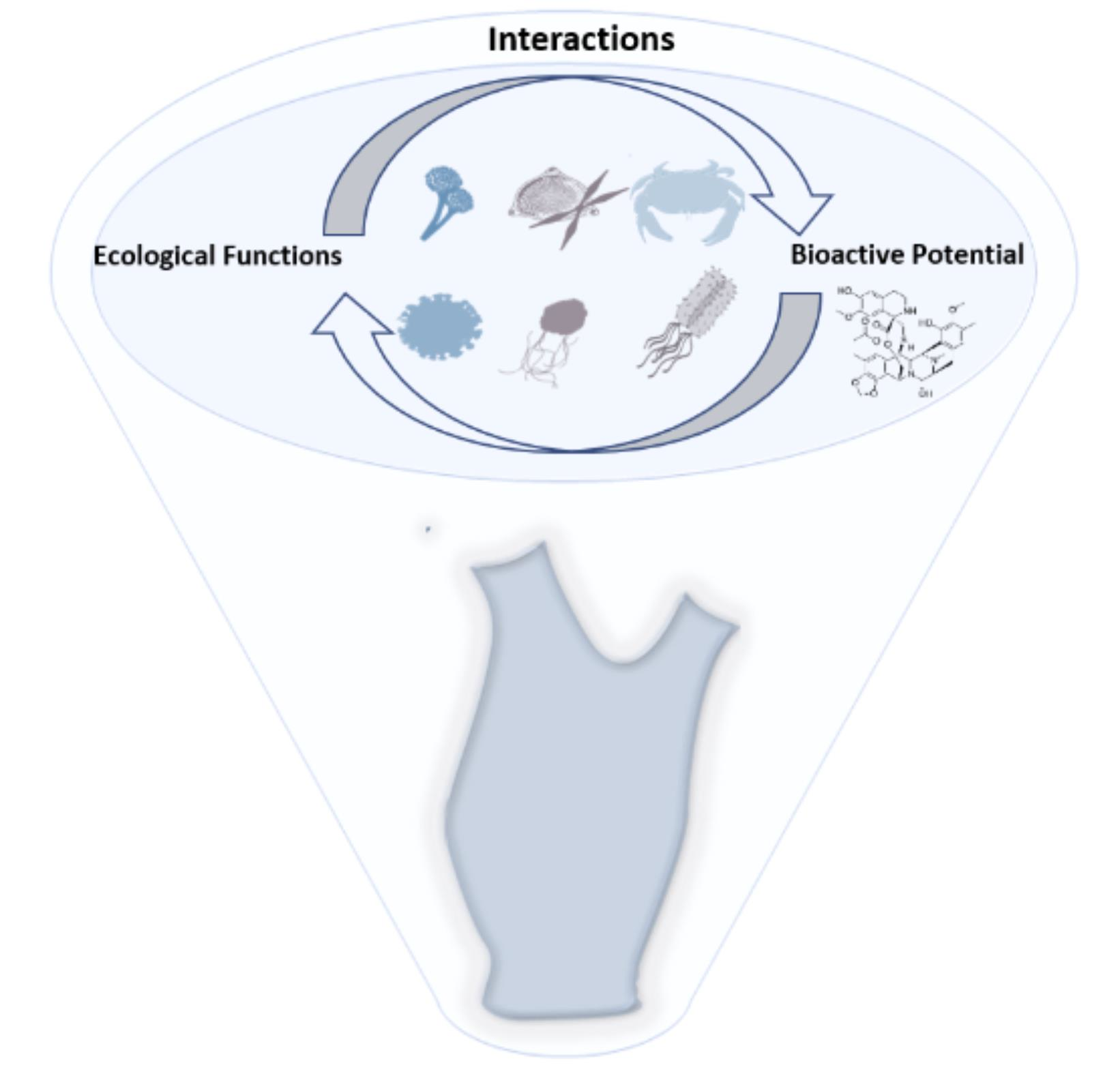The textbook-style illustration features a pastel-rendered image, framed by a lightbulb-shaped blue border that is narrow at the bottom and rounded at the top. The central focus of the image is an inverted cone, its bottom resembling a simplified heart valve or a fragment of an aorta, outlined in blue. Above this is an ellipse-shaped text box with a light blue background and border, labeled "Interactions" in bold, black font. Inside the ellipse, the left side is labeled "Ecological Functions" and the right side "Bio-active Potential".

Two elongated arrows create a clockwise circular motion around the ellipse, depicting a cycle. Various ocean creatures such as crabs, jellyfish, and possibly sea urchins and other small sea critters are illustrated within this cycle. These illustrations surround a central chemical diagram with hexagonal shapes and various elemental labels indicating chemical structures, though the fine details are too small to read clearly.

Below the "Bio-active Potential" section, a detailed chemical diagram is present with hexagon shapes and element labels. Adjacent to the "Ecological Functions" section, the drawing includes various oceanic organisms and other scientific objects like a featureless crab and detailed crustaceans, connected by vertical lines incorporating more fine details like bands and tails.

The overall image serves as an educational diagram explaining the interactions between ecological functions and bio-active potentials, using both textual and visual elements to convey the information.